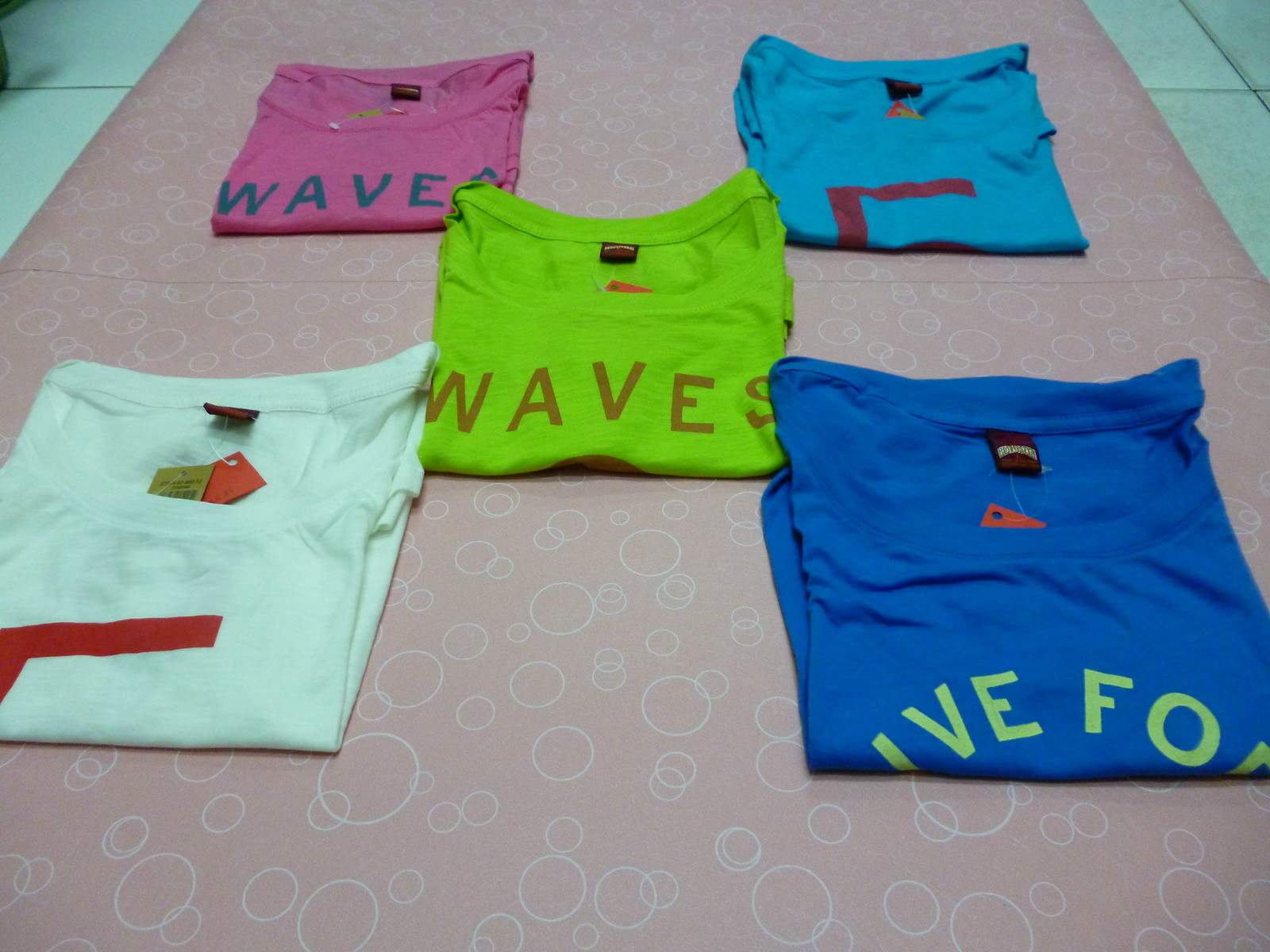The image is a full-color photograph taken indoors, featuring a white tile floor partially covered by a pink mat adorned with overlapping white circles of various sizes. Arranged in a pattern resembling the five dots on a die, five folded t-shirts are positioned on the mat. In the upper left corner, there is a purple t-shirt with the word "Waves" printed on it in blue letters. The upper right corner holds a light blue t-shirt, which partially reveals an upside-down red "L" or potentially a large letter "E" or "F". The center of the arrangement features a uniquely shaded green t-shirt, also bearing the word "Waves". The lower left corner contains a white t-shirt identical to the light blue one in the upper right, complete with a "For Sale" tag. Finally, the lower right corner shows a dark blue t-shirt with green printing that reads "Live For," though the rest of the text is obscured by the fold. The detailed and colorful arrangement of the shirts against the patterned mat creates a visually engaging display.